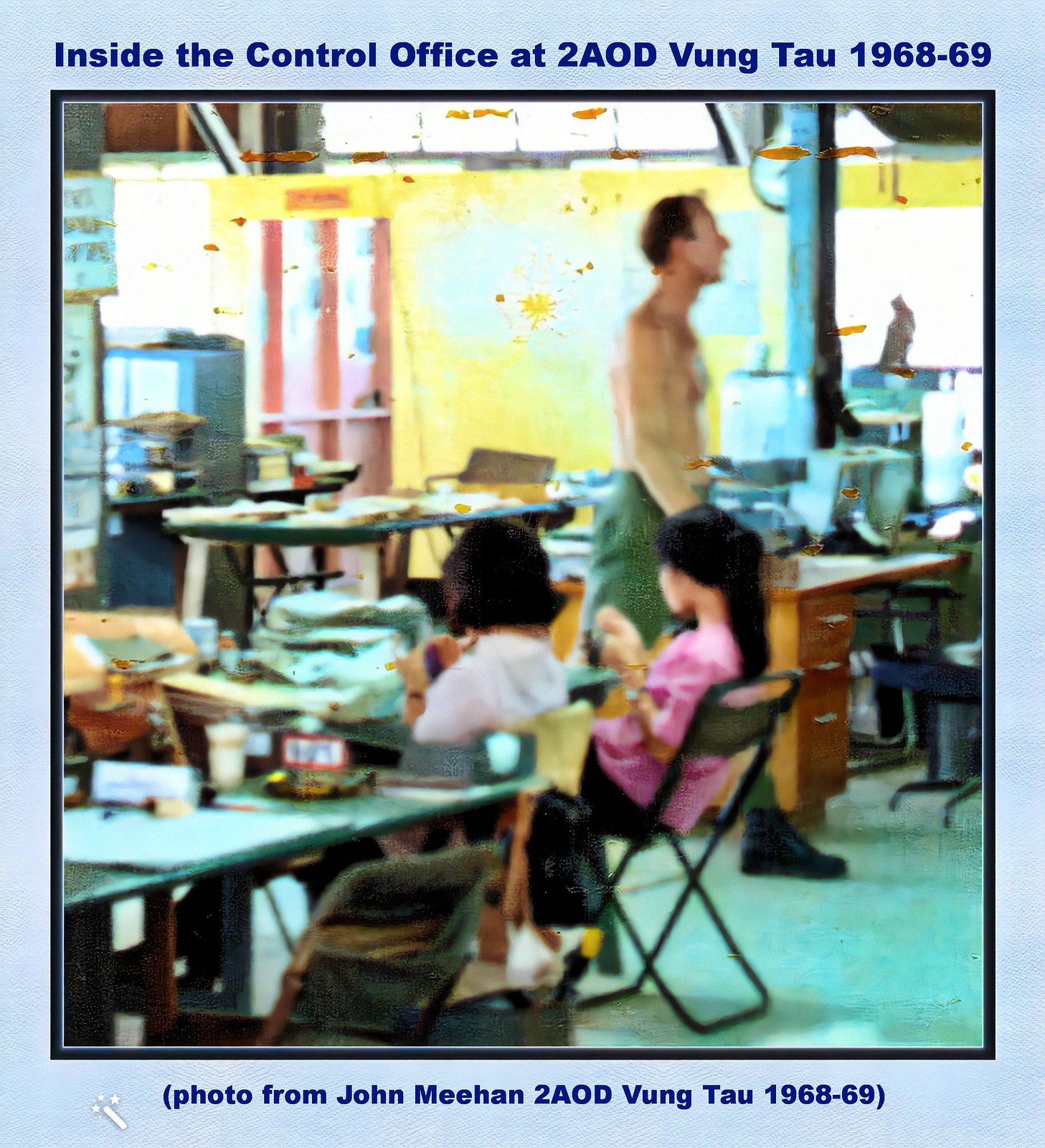The photograph, slightly out of focus and bordered in blue, features a shirtless man with receding light brown hair, in green fatigue pants and black combat boots, standing inside a cluttered control office at 2 A.O.D. Vung Tau, 1968-69. The office space is filled with tables, desks, numerous papers, files, and stationery items. Two women, one in a pink top with long hair and the other in a white top with short hair, sit with their backs to the camera on folding chairs at a desk. At the top of the photo, blue text reads, "Inside the Control Office at 2 A.O.D. Vung Tau, 1968-69," while the center bottom text states, "Photo from John Meehan, 2 A.O.D. Vung Tau, 1968-69." A computer and a computer table are also visible, adding to the scene's period-specific office environment.